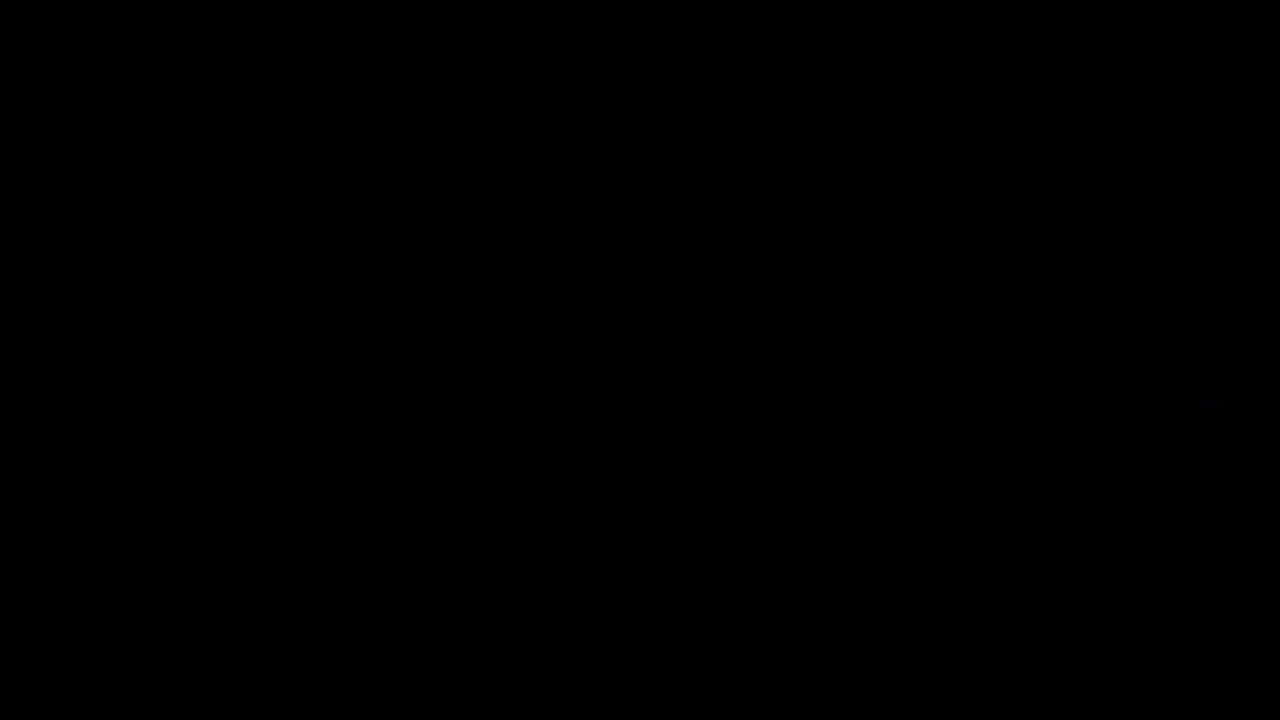This image features a horizontally aligned, solid black rectangle with no interior details, subjects, text, or colors. The image ratio lies roughly between 1:2 and 9:16, emphasizing its rectangular shape. It is simply a large, blank, black rectangle, devoid of any features or elements, representing pure black nothingness.